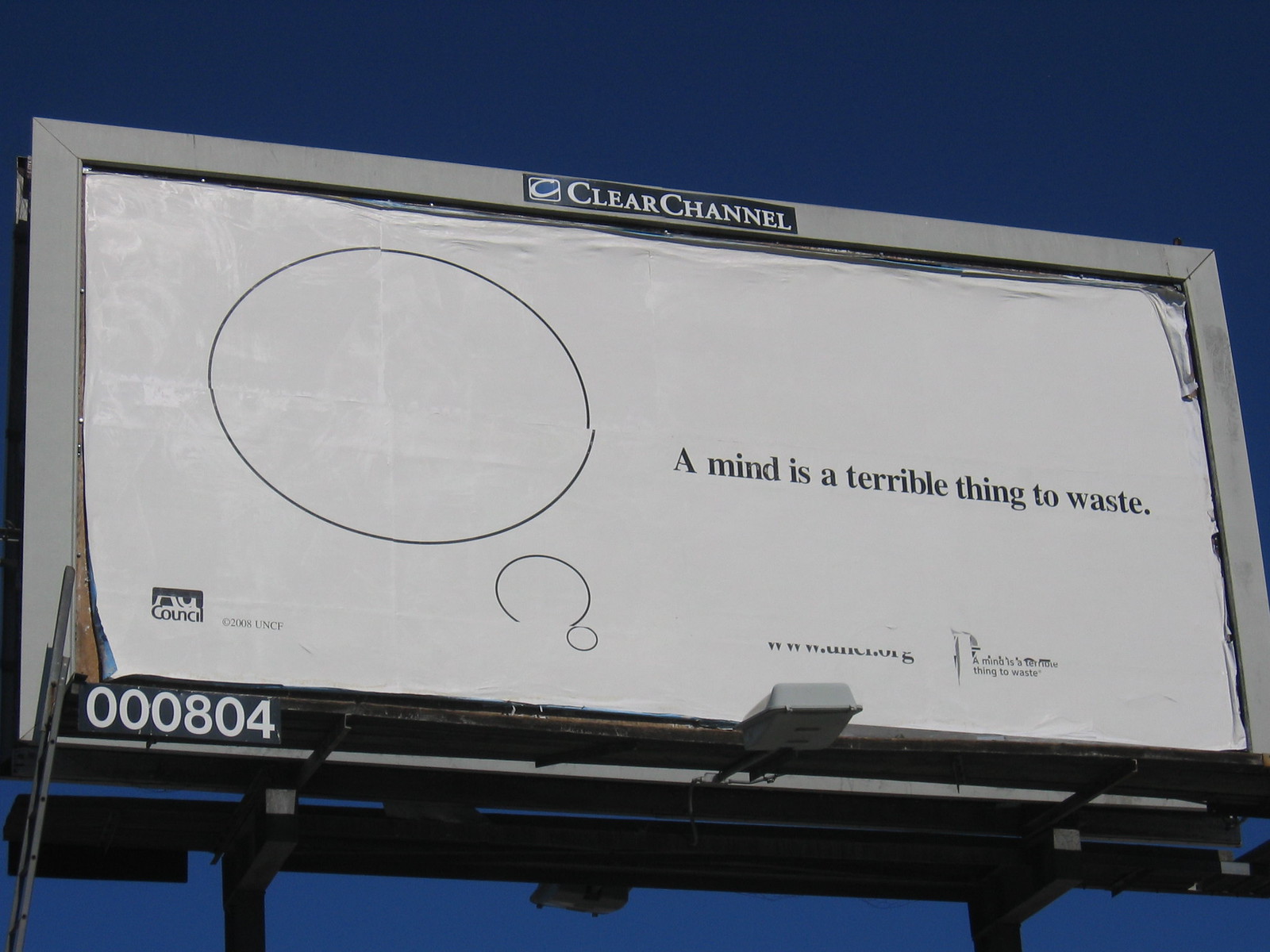The image showcases a close-up, angled view of a rectangular billboard taken from ground level against a dark blue evening sky, suggesting it was taken around 7-8 PM. The billboard belongs to Clear Channel, identified by a logo featuring a white "C" in a square background next to the words "Clear Channel" in white, all contained within a centered black rectangle at the top of the gray-framed billboard. The main content displayed on the billboard is set against a white background with a thinly drawn large black circle, resembling a partial question mark with a smaller circle attached to one edge. Adjacent to the large circle, bold black text reads, "A mind is a terrible thing to waste." Beneath this phrase is smaller black text that’s difficult to discern. On the bottom left of the white area, there is a logo for the Ad Council. The lower left corner of the outer gray frame features white numbers "000804" inside a small black rectangular frame. Additionally, there is a single light attached to the base of the billboard, illuminating the display.